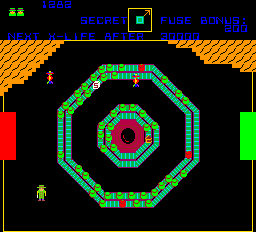This is an image depicting a screenshot from an unidentified video game. At the top of the screen, there's a banner displaying the text "Secret Views" and a "Bonus" indicator. Below this, the player's progress is tracked under a section titled "Life After," showing that the player still has two lives remaining. The main gameplay area features a symmetrical octagonal grid, subdivided into two concentric rows, with two additional, proportionally smaller rows situated at the center. The color scheme incorporates a green grid against a black backdrop, interspersed with rusty-colored elements.